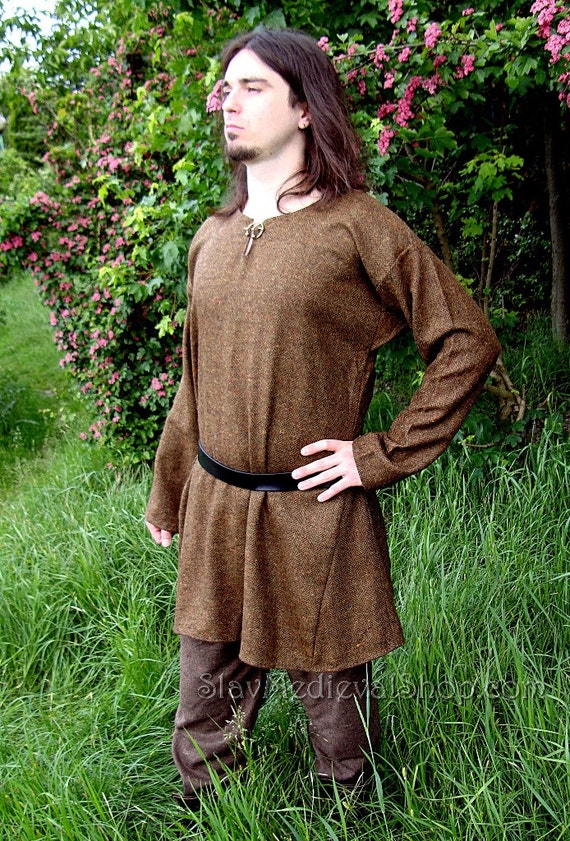The image depicts a white man with shoulder-length dark brown hair and a goatee, standing in a lush, tall grass field. The grass reaches up to his shins, emphasizing its height and vibrant green color. He is dressed in Renaissance attire, including a long-sleeve brown tunic cinched at the waist with a black belt, and dark brown pants, though his shoes are hidden by the grass. The man poses with his left hand on his left hip, gazing thoughtfully to the left, exuding a serious demeanor. Behind him, there are shrubs adorned with pink flowers and a glimpse of a blue sky in the upper left corner. A watermark at the bottom reads "slavmedievalshop.com".